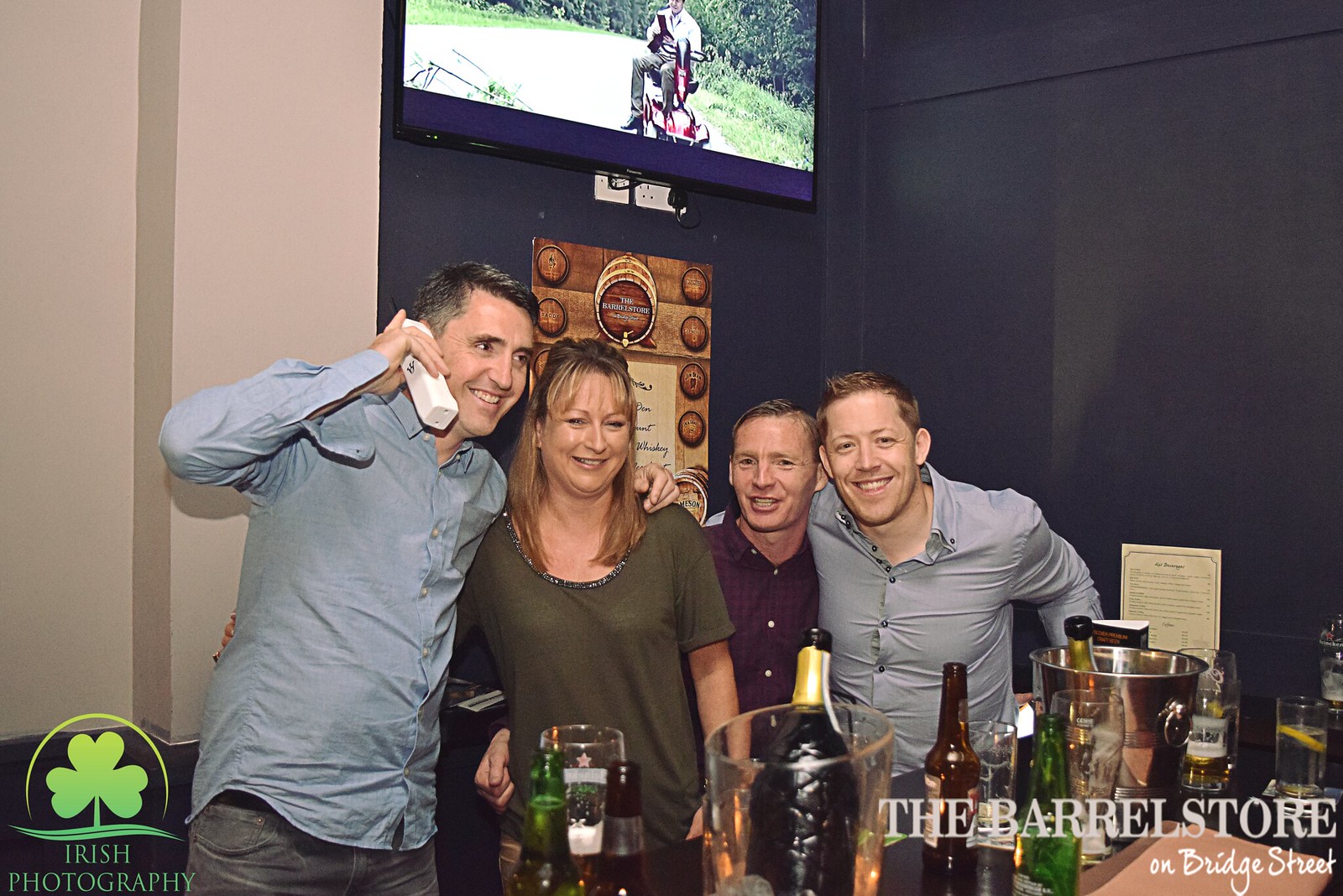This landscape image depicts four people standing behind a bar counter in a room with distinct navy blue and white walls. Positioned from left to right, the first man wears a long-sleeved blue button-down collared shirt while holding a phone to his ear and smiling directly at the camera. To his right, a blonde woman in a green bejeweled scoop neck shirt also smiles at the camera. Next, a man in a purplish button-down collared shirt shares a smile with the viewer, while the final man on the far right, clad in a blue button-down collared shirt, joins in the cheerful pose. The individuals are interlocking arms around each other’s shoulders, conveying a sense of camaraderie and joy. Above them is a television screen displaying an image of a man on a scooter. Situated behind them, there's also a poster adding to the cozy ambiance of the scene. In front of the group, the bar counter is adorned with various bottles, further suggesting a festive environment. In the lower left-hand corner, a green shamrock icon accompanied by the text "Irish Photography" is visible, and in the lower right-hand corner, it reads "The Barrel Store on Bridge Street," indicating the location.